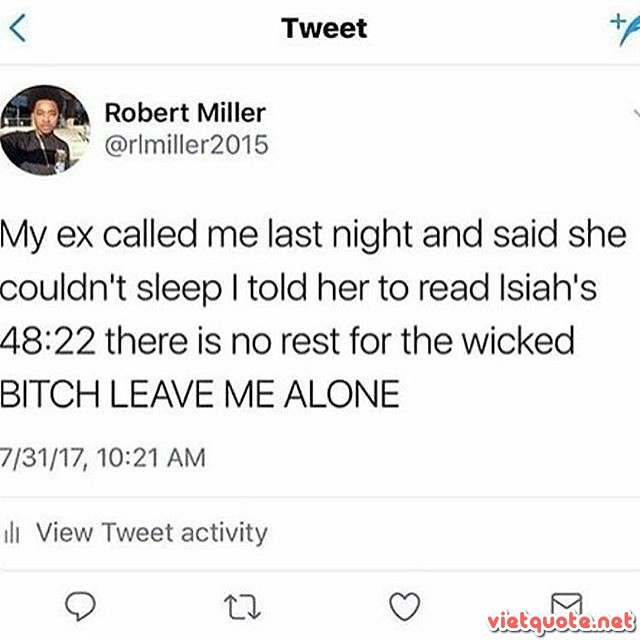This is a detailed screenshot of a tweet posted by Robert Miller (@rmiller2015) on July 31, 2017, at 10:21 a.m. The tweet features a profile image of a young Black man and reads: "My ex called me last night and said she couldn't sleep. I told her to read Isaiah 48:22, 'There is no rest for the wicked.' BITCH, LEAVE ME ALONE." The interface indicates it was taken from an app, with a back arrow icon visible in the top left corner. At the bottom of the tweet, options for viewing tweet activity, commenting, retweeting, liking, and a quill icon are present. An orange text link to VietQuote.net appears in the lower right-hand corner.